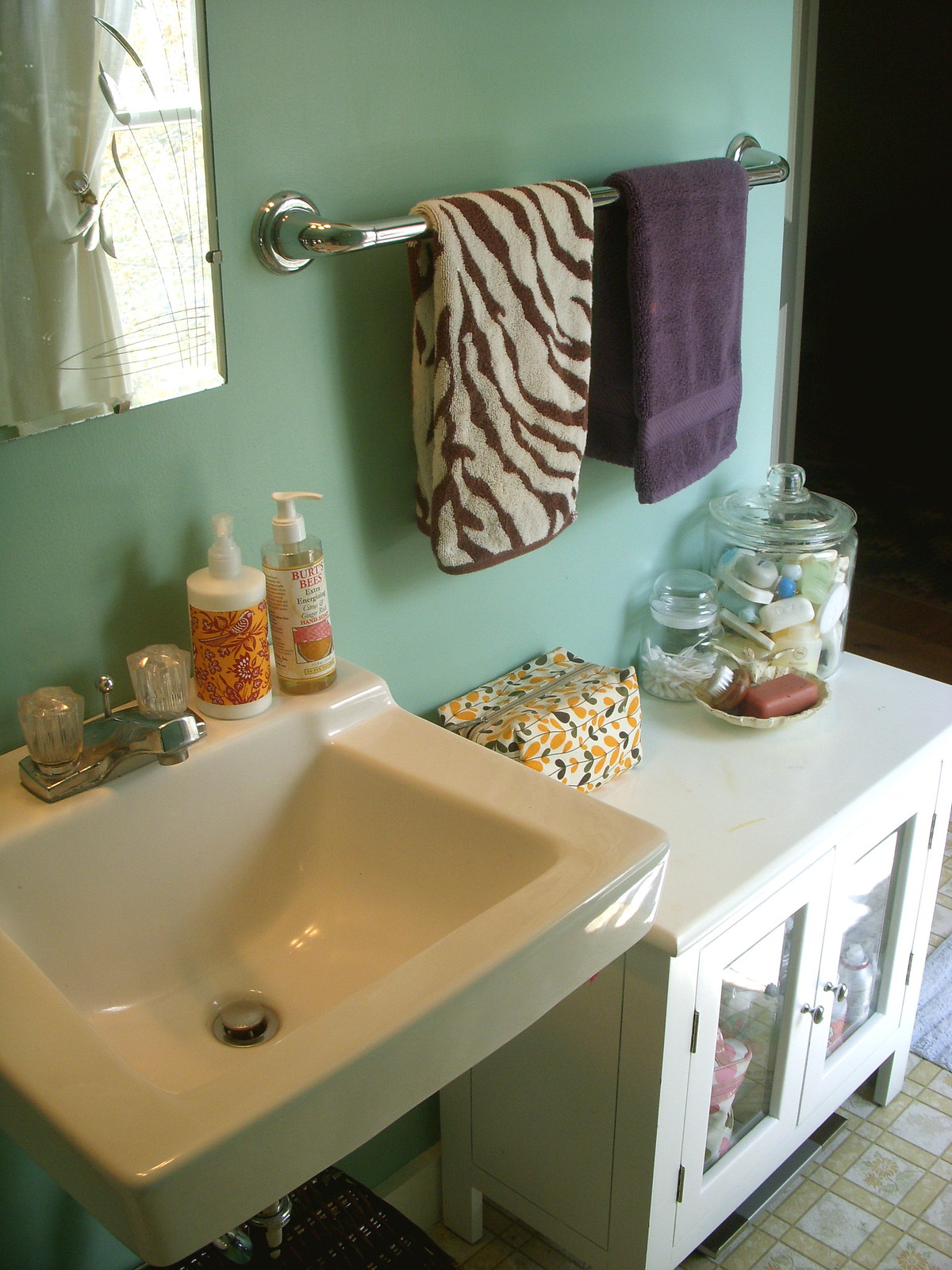The image depicts a bathroom with a predominantly mint green color scheme on the back wall. On the left side, there's a mirror that appears to be part of a medicine cabinet, reflecting an open window with curtains drawn back, allowing ample natural light into the room. 

To the right of the mirror, a silver towel bar holds two towels: a white towel with black stripes on the left and a purple towel on the right. Below the mirror, there's a white porcelain sink featuring a silver drain and crystal handles on both sides, with a silver spout in the center. 

On the right side of the sink, there's a white bottle of soap with an orange and red label and a cap. Next to it, another bottle with a "Burt's Bees" label is equipped with a pump. Further to the right, there's a decorative container or bag adorned with yellow and blue leaves. Next to this, a large jar containing various soap parts and a separate jar of Q-tips can be seen.

Underneath the sink, a cabinet with glass doors offers a glimpse of the contents stored inside. The floor is tiled, featuring a pattern of white squares with either white or yellow bars running through them.